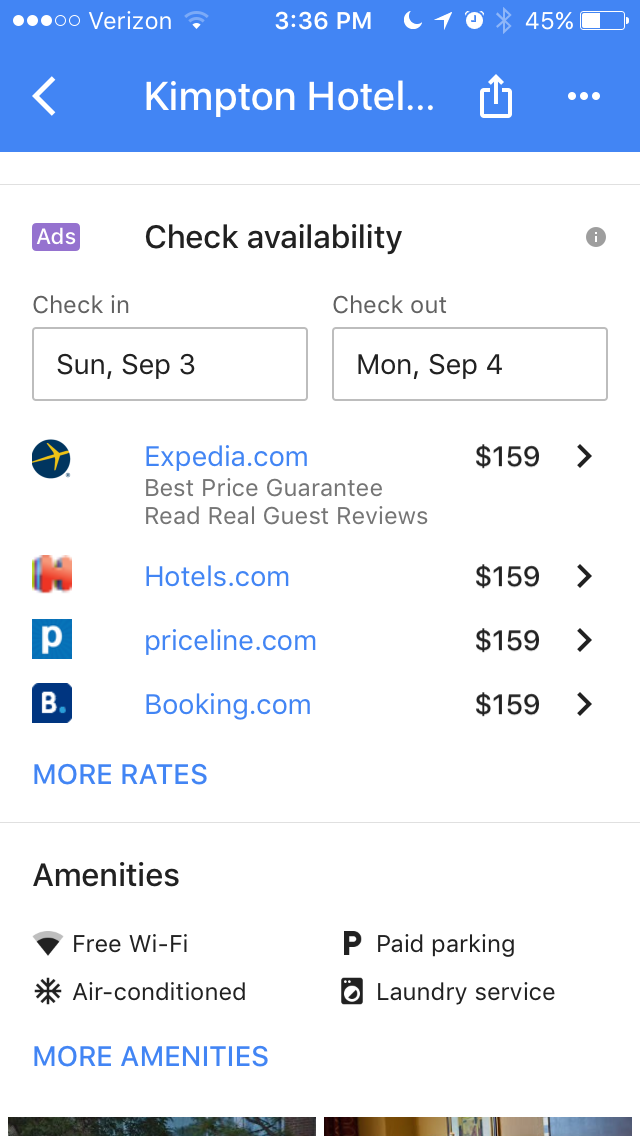This image, captured on an iPhone with a 45% battery life and the time displayed as 3:36 PM, appears to show a hotel booking interface for the Kempton Hotel. The iPhone is set to silent mode and the network provider is Verizon.

Encased in a blue box at the top of the screen, the hotel information suggests users can check availability below. On a white background, a purple box labeled "Ads" follows the availability check option. Next to "Check Availability," there's a small eye icon inside a gray circle.

The interface allows users to input their check-in and check-out dates, specifically showing a check-in on Sunday, September 3rd, and a check-out on Monday, September 4th. Below this, several booking options are listed:
- Expedia.com with a best-price guarantee and real guest reviews, priced at $159.
- Hotels.com with the same rate of $159.
- Priceline.com, identified by a prominent "P," at $159.
- Booking.com, marked by a large "B," also at $159.

A "More rates" option is highlighted in blue, set apart into its distinct section. Following this, amenities are listed with corresponding icons, including free Wi-Fi, air conditioning, paid parking, and laundry service. There's also a "More amenities" option in blue, although part of the associated text is cut off, leaving some details obscured.

The images and the rest of the content appear truncated at the bottom edge, suggesting the full details are not fully visible in this screenshot.